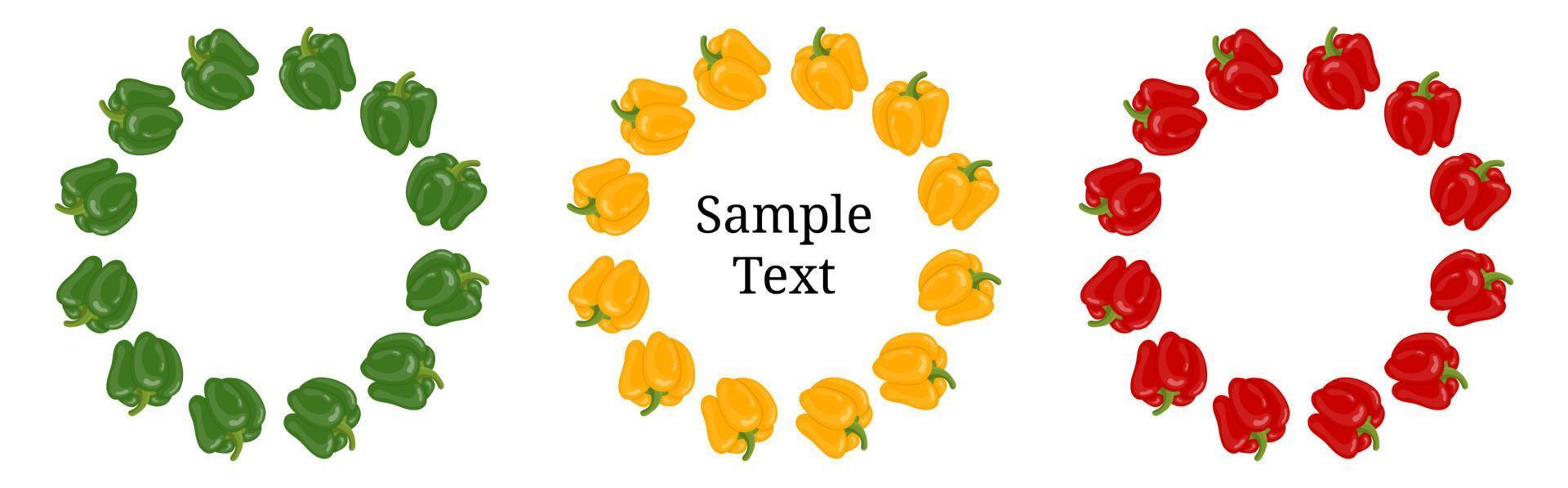The image features a stark white background with three distinct rings of illustrated bell peppers, arranged side by side. The leftmost ring comprises about 12 green bell peppers, each with a green stem. In the center, another ring of 12 yellow bell peppers with green stems forms a circle, and within this circle, the words "sample text" are printed in black. To the right is a third ring made up of 12 red bell peppers, all of which also have green stems. The layout creates a visually balanced and colorful template, possibly intended for use in graphic design or as an internet meme.